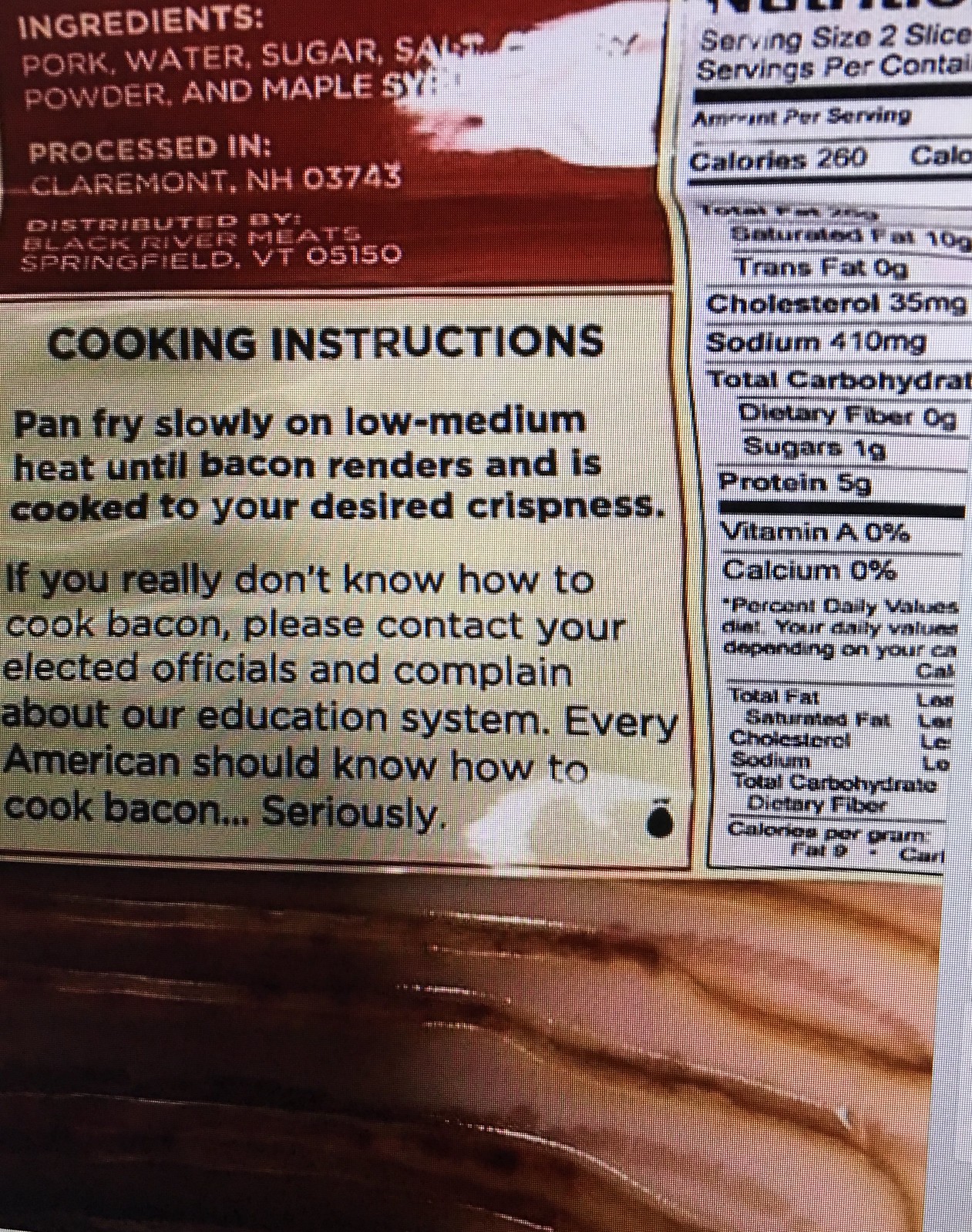The image is a close-up shot of the back side of a bacon package, captured off a digital screen. The top segment of the package displays the ingredients list, which includes pork, water, sugar, salt, celery powder, and maple syrup. Some of the text is obscured by a white patch. The bacon is processed in Claremont, New Hampshire, 03743, and distributed by Black River Meats, Springfield, Vermont, 05150, with this information displayed in white text on a red background. The cooking instructions below advise pan frying the bacon slowly on low-medium heat until it renders and reaches the desired crispiness, humorously suggesting that anyone who can't cook bacon should contact their elected officials to complain about the education system. The nutritional facts are partially visible, showing a serving size of two slices and 260 calories. The image captures part of the bacon slices behind the plastic, with a shadow on the left and clearer visibility on the right.